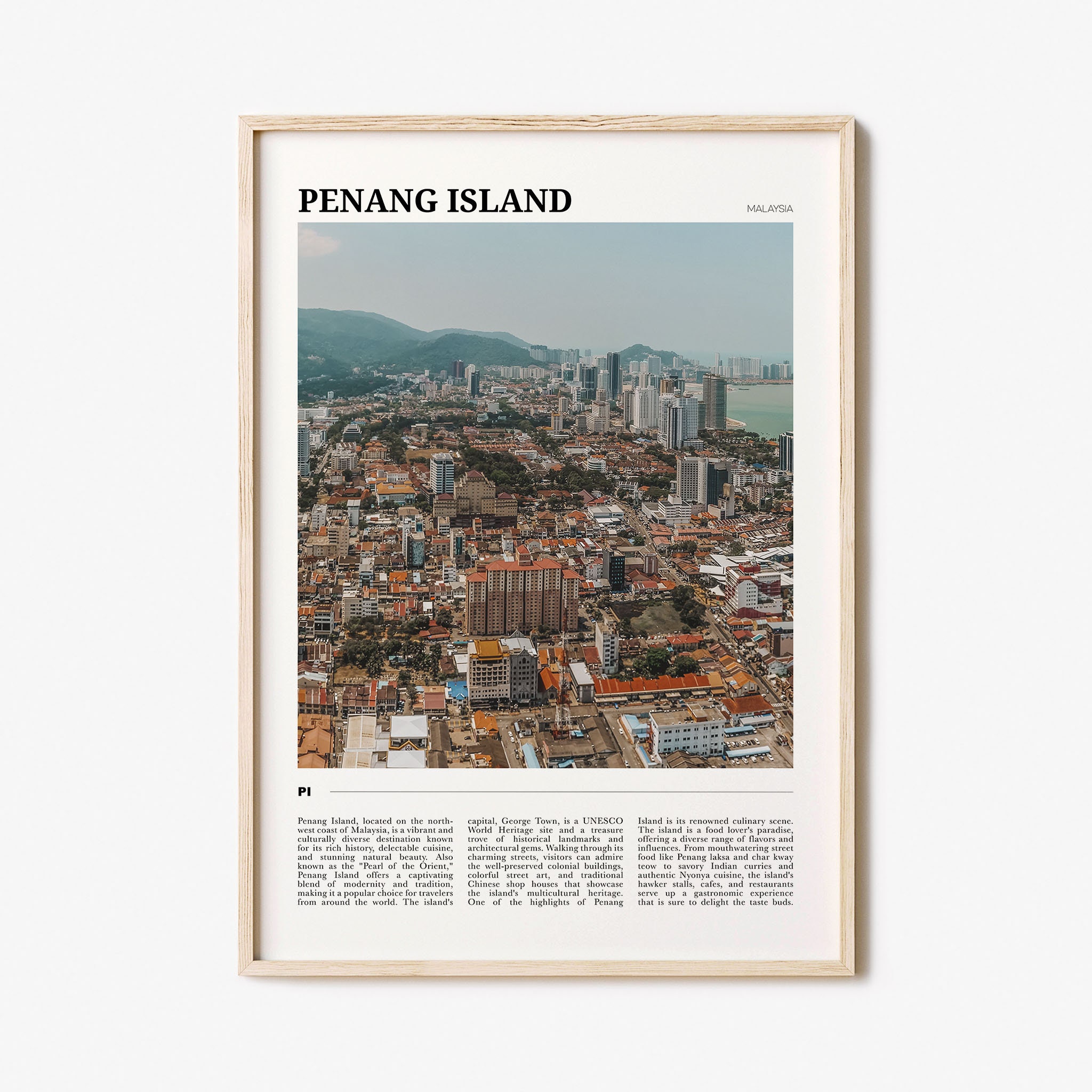The image features a color photograph of a densely populated city, identified as Penang Island, Malaysia. The photograph is encased in a thin, light wooden frame of an oblong shape, hanging on a white wall. At the top of the image, "Penang Island" is written in large black letters, and "Malaysia" appears on the right side. The cityscape, presented from an aerial viewpoint, reveals a bustling metropolis with numerous tall buildings in the foreground and a mix of lower houses. In the background, Blue Mountains rise on the left, while an expanse of ocean is visible to the right. At the bottom of the frame, there are three paragraphs of text that describe Penang Island as a vibrant and culturally diverse destination situated on the northwest coast of Malaysia. The text highlights the island's rich history, delectable cuisine, and stunning natural beauty, referring to it as the Pearl of the Orient. The overall layout features the photograph centered against a white background, with the descriptive text in three columns at the very bottom.